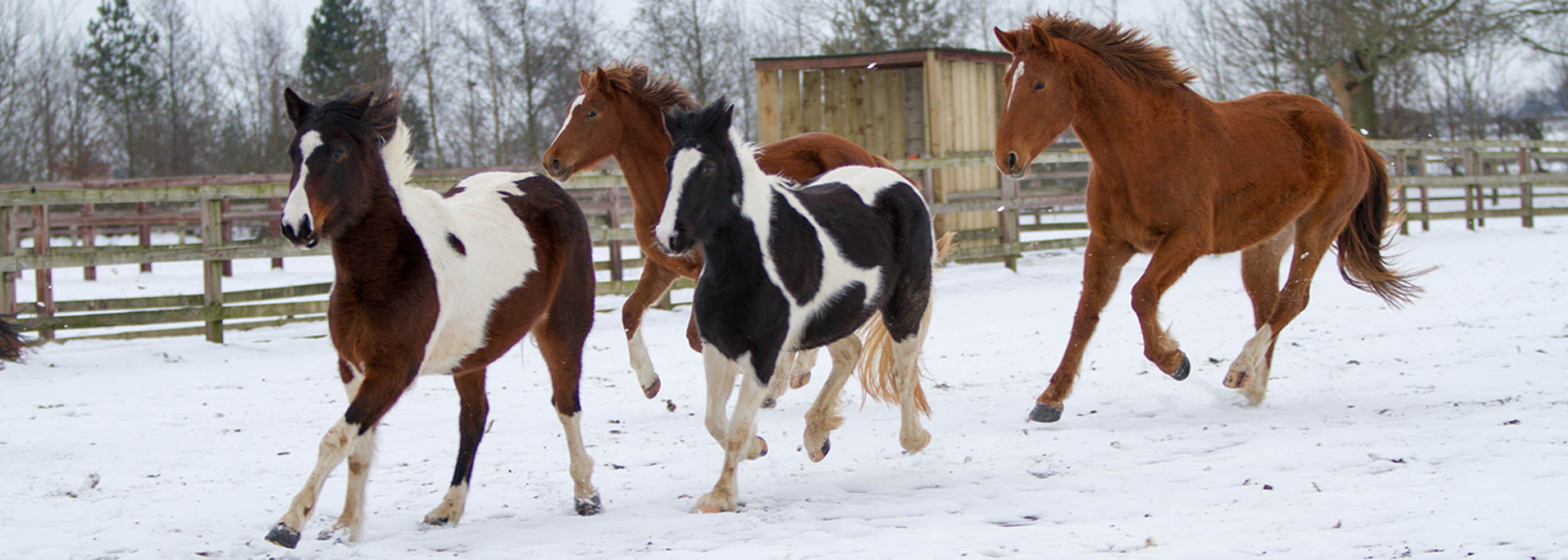The image captures a winter scene featuring four horses running to the left across a snowy, enclosed area. Leading the pack, there are two smaller horses with distinct color patterns: one is brown and white with some black spots, and the other is black and white. Behind them, two larger horses, both a rusty chestnut color with white markings on their faces, follow closely. The ground is covered in snow with a few patches of grass peeking through, indicating cold weather. The background is dominated by trees and includes a small wooden shack. A wooden fence, typical for horse enclosures, runs parallel to the action, while the sky above is overcast, filled with clouds but no snowfall. The horses' thick coats suggest they are well-adapted to the winter conditions.